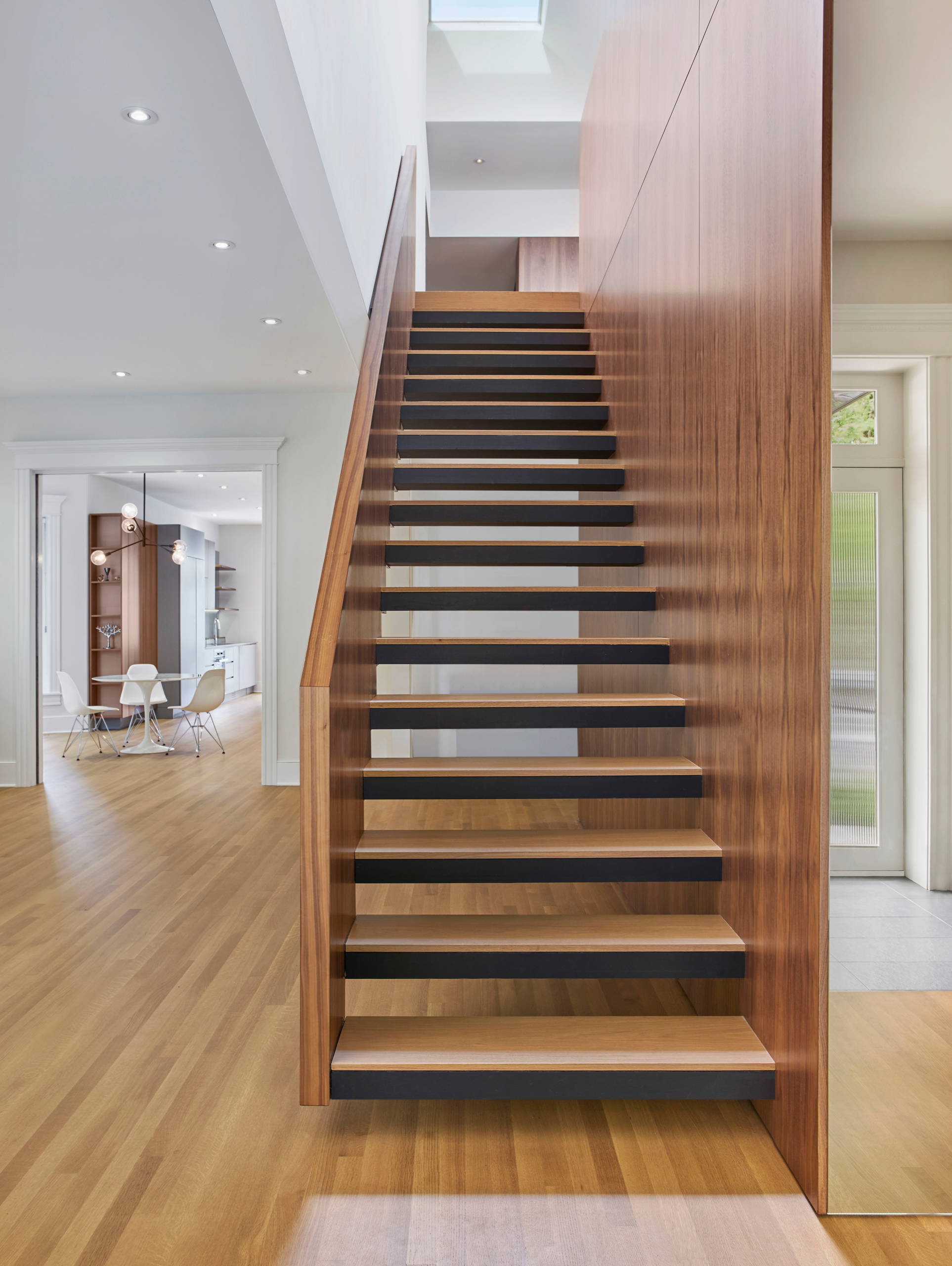The image showcases a sleek and modern interior of a house with a vertically oriented photograph emphasizing the centerpiece—a beautifully crafted brown wooden staircase. This unique, open-step design allows visibility through the steps, contributing to the spacious feel of the home. The staircase is bordered on the left by a large open room and on the right by a full-sized white wall. The surroundings feature white walls and ceilings that accentuate the minimalist and clean design of the house, with shiny wood floors adding a touch of warmth.

In the background, a sophisticated dining area is visible, furnished with a white table and white chairs, indicative of a kitchen or breakfast nook. This dining area is illuminated by a striking modern chandelier with rounded lights. Additionally, there is a textured glass door on the right side of the staircase, offering a glimpse of green plants outside and enhancing the natural light within the space. The overall atmosphere is very elegant, modern, and well-lit, highlighting both the craftsmanship of the staircase and the airy, contemporary design of the home.